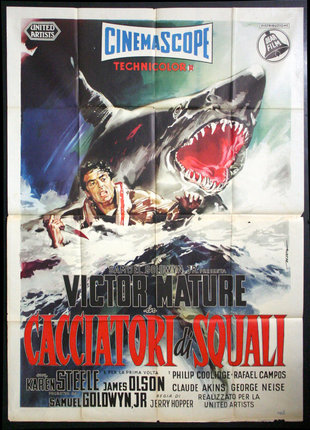This image depicts a vintage movie poster featuring a thrilling scene dominated by a menacing black shark lunging out of the water, its gaping red mouth revealing sharp white teeth. The background contrasts with its dramatic elements by showcasing a striking green sky. A distressed man with a life preserver around him struggles in the foamy waves; in one hand, he clutches a bloody knife. The poster, visibly worn and folded into squares, includes a prominent white border. At the top, 'Cinemascope' is displayed in a blue, curved rectangle, followed by 'Technicolor' in red, and 'United Artists' positioned in the upper left corner. The upper right corner bears a partially obscured logo reading '...something film.' Below the water scene, the red text announces 'Victor, Mature, Kasiatori Di Squali', with 'Victor, Mature' in black, tying in additional names in black underneath. All these elements together create a vivid and intense advertisement for an action-packed film, captured in the nostalgic style of vintage movie posters.